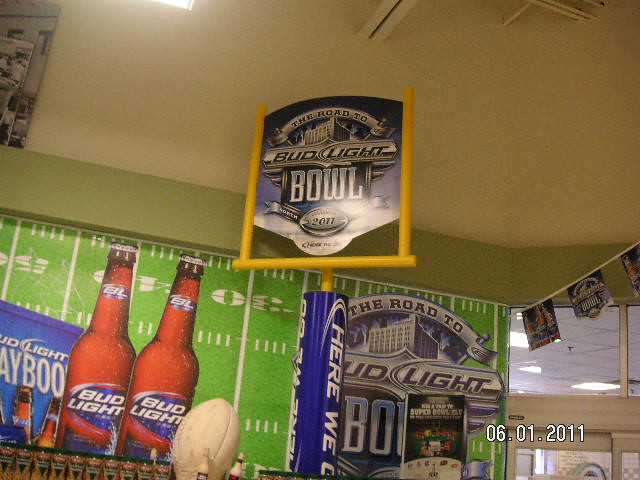The photograph, taken on June 1, 2011, captures an indoor setting, likely within a bar or store. The ceiling is ivory with white beams, and the upper left corner features a light fixture and what appears to be a mirror or poster. Below the ceiling is a green border on the walls. Dominating the scene is a vibrant advertisement for the Bud Light Bowl. Central to the display are golden goalposts with a padded blue base, bearing the slogan "Here We Go" and a sign that reads "Bud Light Bowl 2011." This is complemented by a depiction of a football field, complete with marked lines and two prominently displayed Bud Light bottles. In the backdrop, there is also a "Bud Light Playbook" graphic. The entire setup suggests an event or promotion celebrating the Super Bowl, sponsored by Bud Light.